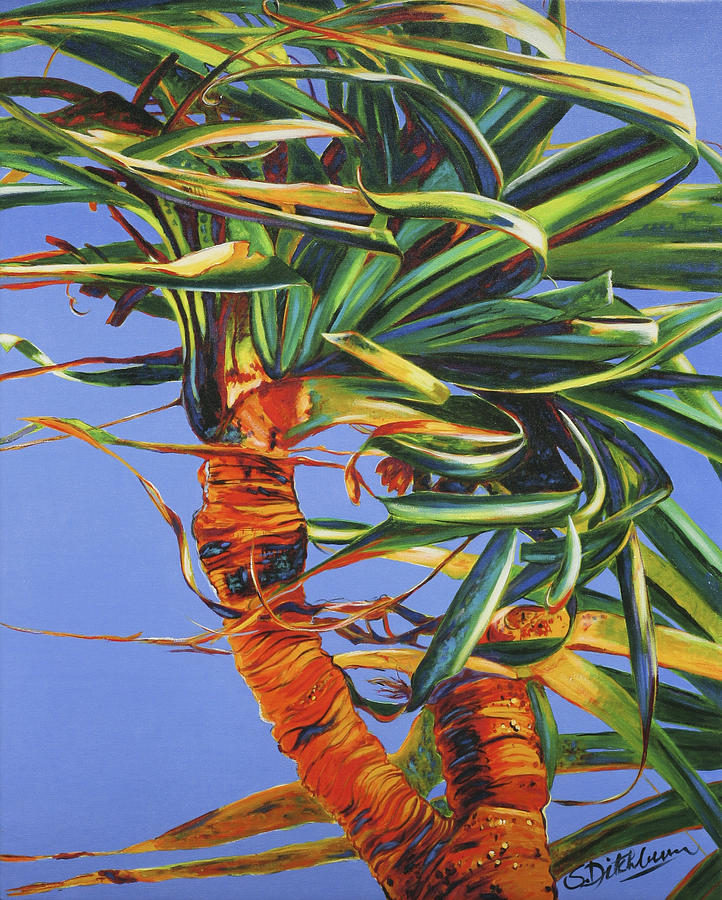The image provided is a vibrant and colorful painting that prominently features a single tropical tree, likely a type of palm tree, against a light blue backdrop. The tree's trunk rises and splits into two branches: one that extends straight upward, and another that curves slightly to the left. At the top of these branches, thick and long green leaves stand out, bending backward to the left as if blown by the wind. The leaves and branches take up the entire upper half of the painting.

The painting incorporates a diverse palette, including shades of green, yellow, red, orange, maroon, black, and blue, making it visually striking and emphasizing the lively, dynamic scene. Despite the vibrant colors, the focus remains solely on the tree, with no other objects present in the composition.

In the bottom portion of the painting, specifically in the right corner, there's a signature, although it's difficult to read. The painting is well-lit and detailed, capturing the essence of this tropical tree as if portrayed in the wild during a bright day, highlighting its natural beauty and movement.